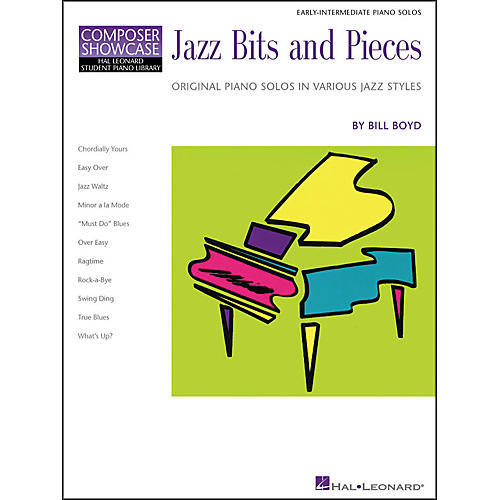This image represents a vibrant book cover designed for early intermediate piano students. Dominating the cover, the title "Jazz Bits and Pieces" is elegantly displayed in a stylish purple font, hinting at the jazz influence within the pages. Positioned at the top right-hand corner, the text "Early Intermediate Piano Solos" denotes the skill level targeted by this collection.

In the top left-hand corner, albeit in a relatively small font, the label "Composer Showcase Leonard Student Piano" is seen, with "Composer Showcase" distinguished in purple. Beneath the main title, a descriptive subtitle reads, "Original Piano Solos in Various Jazz Styles," providing further insight into the content's genre and variety. 

The author, Bill Boyd, is credited prominently, ensuring recognition for his work. Along the left side of the cover, the names of included pieces are listed: "Cordially Yours," "Easy Over," "Jazz Waltz," "Minor a la Mode," "Must Do Blues," "Over Easy," "Ragtime," "Rockabye," "Swing Ding," "True Blues," and "What's Up." 

A green square features a piano illustration, adding a visual touch that hints at the musical journey within the book.